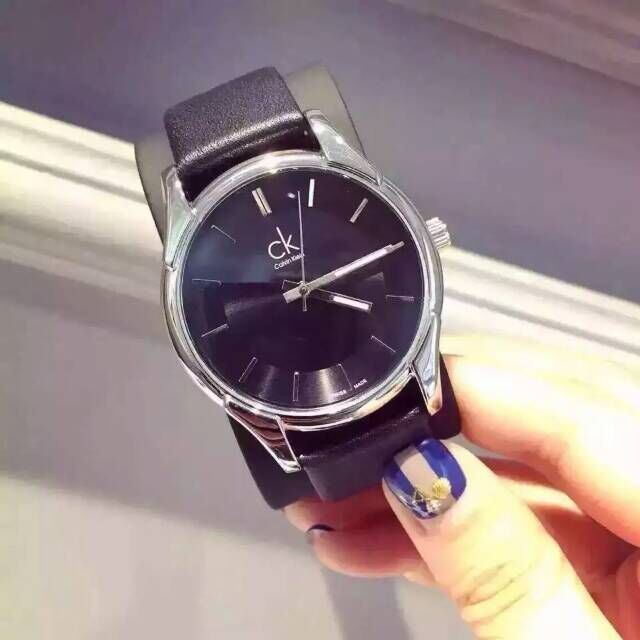A detailed photograph captures a black Calvin Klein wristwatch held by a person's right hand. The thumb, adorned with blue and white striped nail polish accompanied by intricate flower designs, is prominently shown. The watch face, encased in shiny chrome or stainless steel, is sleek with no numbers—only white lines marking the hours, except for the 12, which is denoted by two vertical dashes. The time displayed is a quarter past four and four seconds, with three white hands indicating the hours, minutes, and seconds. The watch band is a combination of shimmering black material and glossy chrome, complementing the minimalist yet sophisticated design. To the right side of the watch, a silver knob is visible. The background features a gray surface with a white border, possibly a wall or countertop, adding a neutral backdrop that highlights the elegant watch and the detailed nail art of the person holding it.